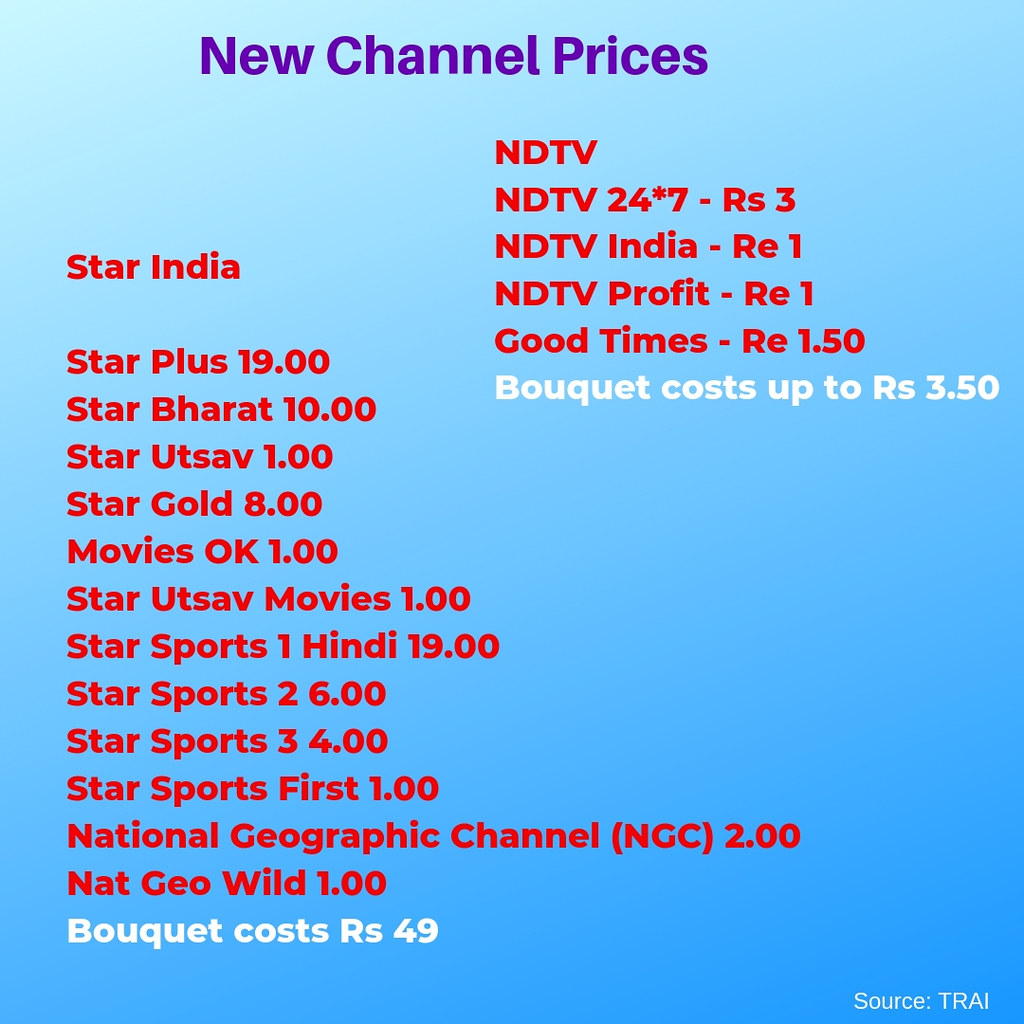The image features a light blue background with a title in purple at the top that says "New Channel Prices". Below the title, in red letters, a list of various channels and their respective prices is shown. Highlights include:

- Star India Star Plus at ₹19.00,
- Star Bharat at ₹10.00,
- Star Utsav at ₹1.00,
- Star Gold at ₹8.00,
- Movies OK at ₹1.00.

It also mentions NDTV 24-7 priced at ₹3.00, NDTV India at ₹1.00, NDTV Profit at ₹1.00, Good Times at ₹150.00, and several Star Sports channels with various prices, including Star Sports 1 Hindi at ₹19.00 and Star Sports First at ₹1.00.

At the bottom, in white letters, it states "Bouquet costs RS 49" and "Bouquet costs up to RS 350". In the bottom right corner, it cites the source as TRAI. The overall layout is neatly organized with distinct column separations, further emphasizing the pricing details.